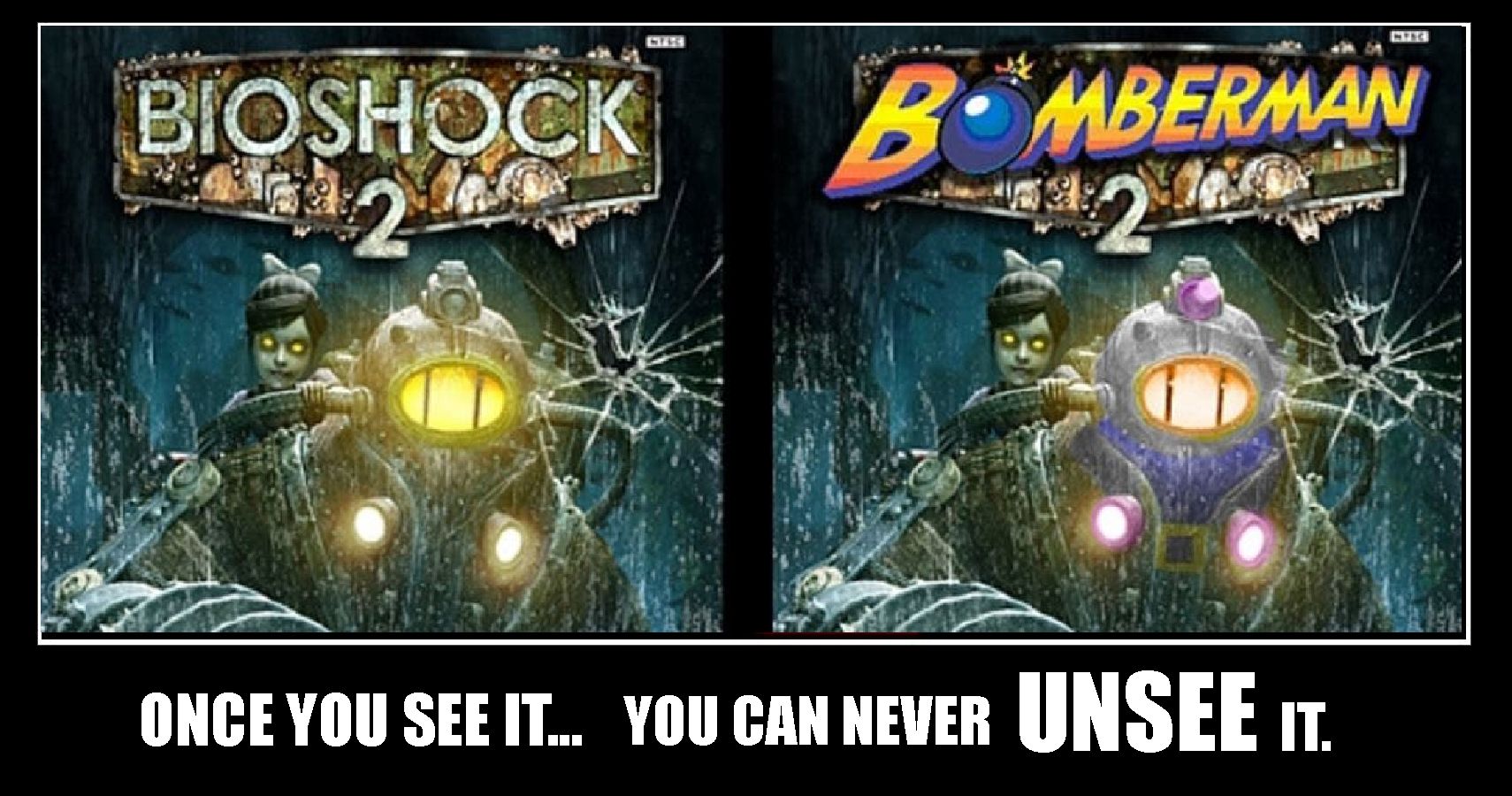The image, set against a black background, is split into two sections each labeled at the top—"Bioshock 2" on the left and "Bomberman 2" on the right. Both sections showcase a strikingly similar picture of a zombie-like girl with light green skin, black hair adorned with a white bow, and glowing yellow eyes, riding a motorcycle. Next to her in each image is a robot-like creature with an oval-shaped light on its front. In the Bioshock 2 section, this light glows yellow, while in the Bomberman 2 section, it has an orangey hue mixed with purple lights. The text at the bottom of the image, rendered in an impact font with the word "UNC" notably larger, reads: "Once you see it, you can never unsee it," emphasizing the eerie and unforgettable nature of the visuals. Each iteration of the girl displays the same annoyed expression, adding to the unsettling atmosphere of the scene.